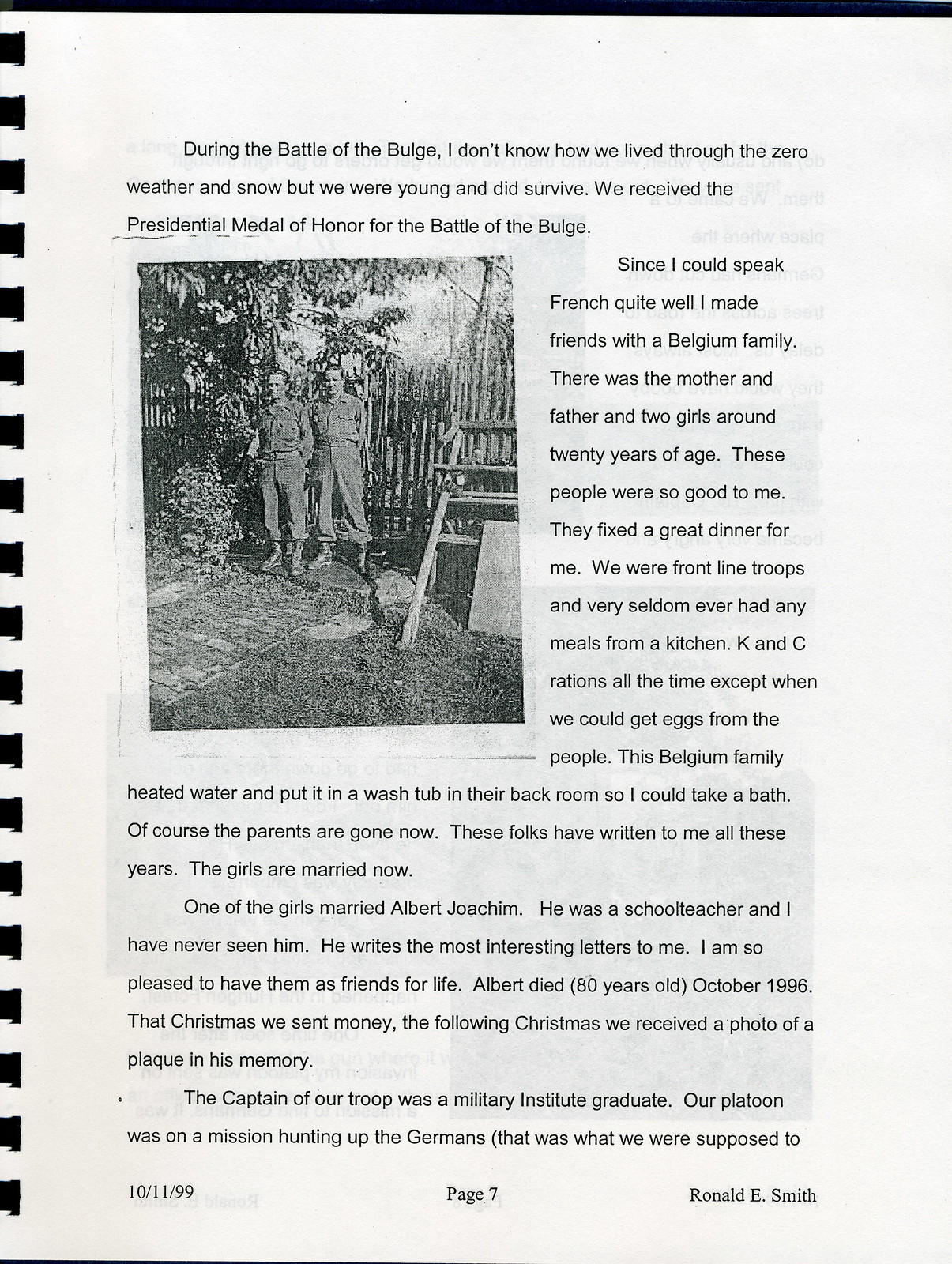The image features a page from a spiral-bound book, likely an autobiography, predominantly comprising text with a monochromatic color scheme of white, black, and shades of gray. The page is dated 10-11-99 in the bottom left corner and marked as page seven in the center at the bottom, with the author's name, Ronald E. Smith, on the bottom right. The central focus is a black-and-white photograph depicting two men in long-sleeve shirts, long pants, and dark boots, standing on a cobblestone sidewalk with grass growing between the stones. Behind them is a wooden picket fence and some trees. The accompanying text narrates experiences from the Battle of the Bulge, mentioning survival through harsh winter conditions, receiving the Presidential Medal of Honor, and forming a bond with a Belgian family. The men recount the kindness of this family, which included parents and two daughters around 20 years of age, who provided a much-appreciated meal. This context sets the scene as part of a reflective wartime memoir.